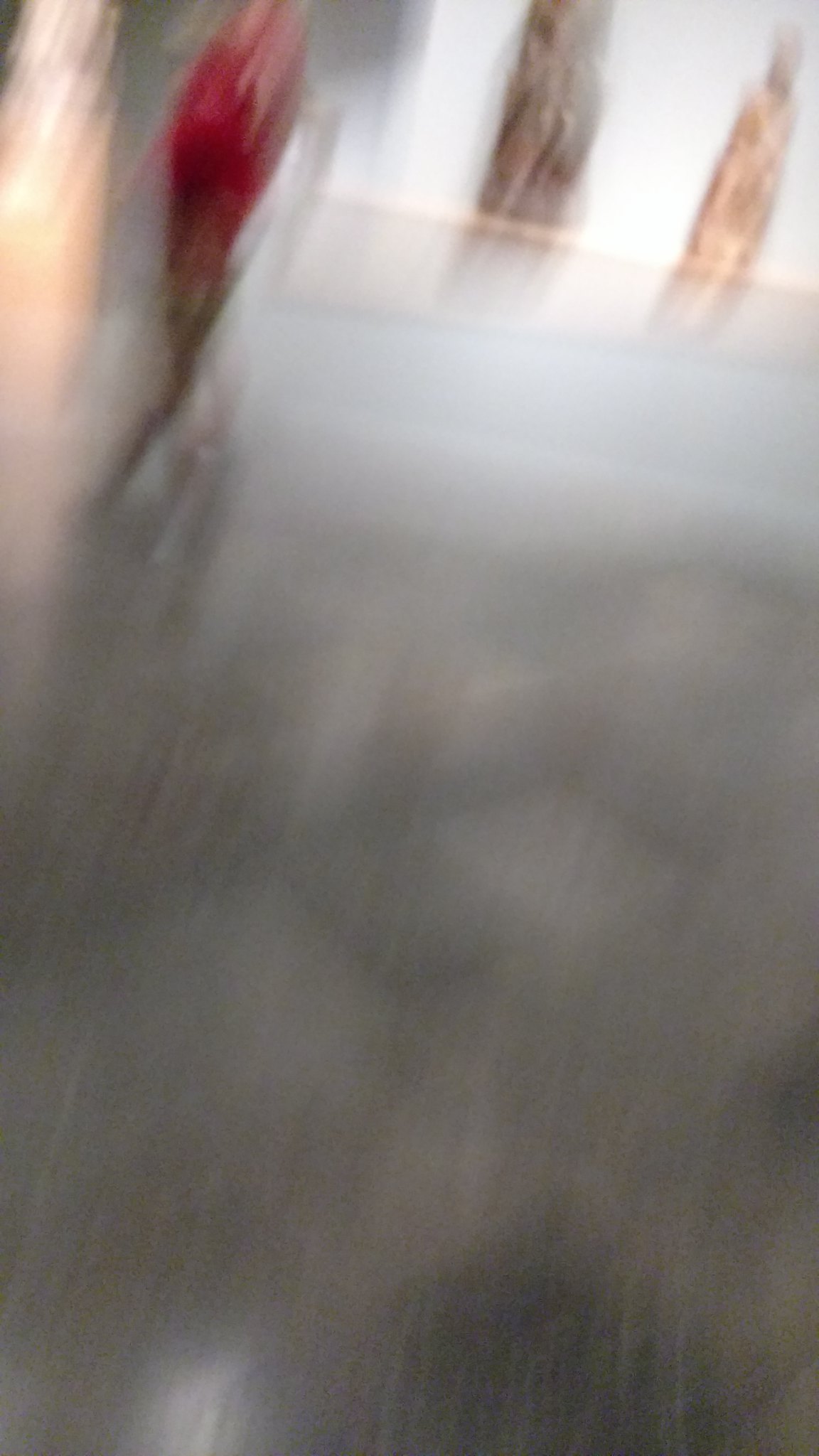This photograph is notably blurry, obscuring much of the detail, particularly in the bottom two-thirds of the image, which appears very gray and shiny, possibly due to rain. In the upper left-hand corner, a woman can be seen walking. She is likely wearing a long-sleeved red shirt and brown pants, with long, blondish hair. The background features a white wall that may belong to a building, adorned with indistinct graphics that might be mannequins or statues. One decorative figure seems brown, and another appears to be gold. The top section of the image includes a series of brush stroke-like streaks in colors ranging from light orange to red, and dark brown to black, with a possible hint of a light brown. Additionally, there's a small yellow line near the right side, which could be an object like a ziplock bag resting on something, although it's difficult to discern due to the blurriness.